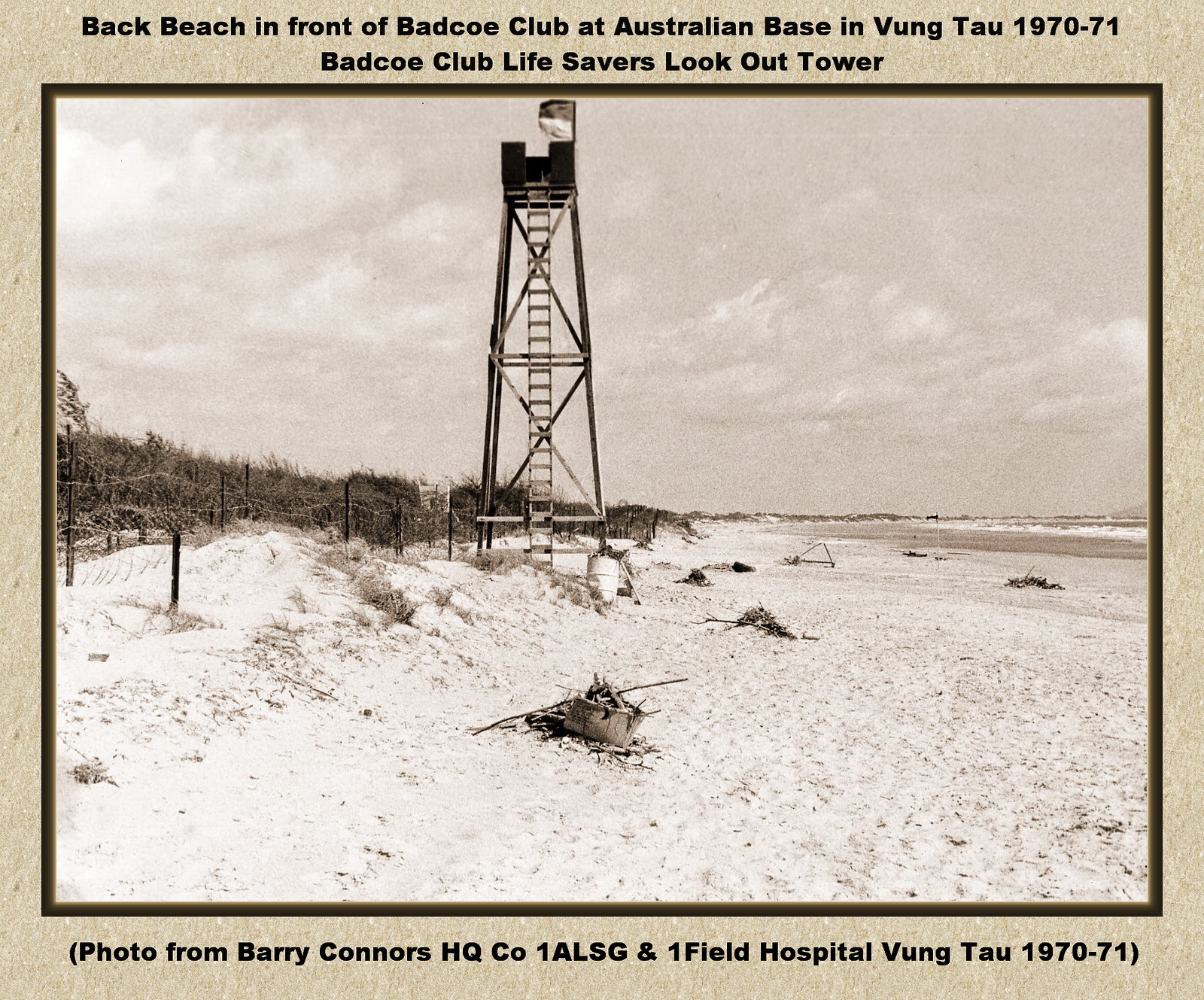The image depicts a black and white photograph of a desolate, old beach with a lifeguard tower. The beach appears barren, with no visible people and sparse, scrubby brush in the background. Sand stretches across the foreground, leading to the ocean on the right side. A wooden lifeguard tower, accessible by a long ladder, stands prominently in the scene. The photo is bordered by a cream-colored frame with black text. At the top of the border, it reads: "Back Beach in front of Badco Club at Australian Base in Vung Tau, 1970-71." Below this, it states: "Badco Club Lifesavers Lookout Tower." At the bottom, it is noted: "Photo by Barry Connors HQ CO 1 ALSG and One Field Hospital, Vung Tau, 1970-71." The sky in the background is overcast with a heavy cloud cover, adding to the overall sense of isolation and abandonment in the picture.